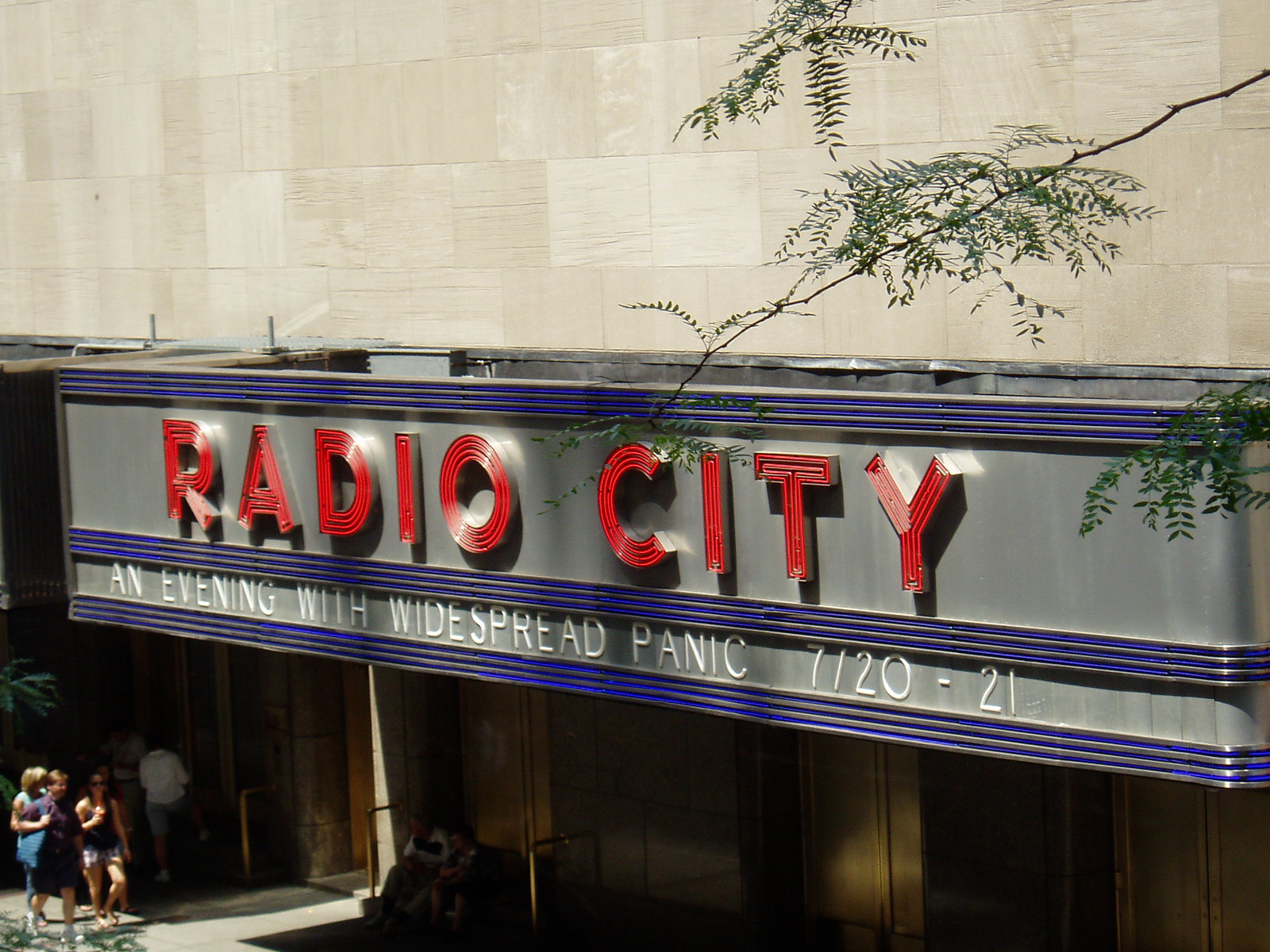This detailed outdoor photograph captures the front of a large building adorned with off-white and tan tiles. Prominently displayed above the entrance is a striking rectangular sign bordered by three lines of blue neon at the top, middle, and bottom edges. The sign's top section, bathed in red neon letters, boldly spells out "Radio City." Below this, in white lettering, it reads "An Evening with Widespread Panic 7/20/21." The sign accentuates golden handles on glass doors beneath it.

Tree branches drape over the building's upper left corner, lending a touch of nature to the urban scene. In front of the building, several people traverse the sidewalk; a group of three adults—two women and a shadowed figure—walk in one direction, while two others move in the opposite direction. Additionally, a stairwell and more doorways are visible on the lower left. This mix of natural and architectural elements, alongside the bustling street life, creates a dynamic and vivid depiction of the location.